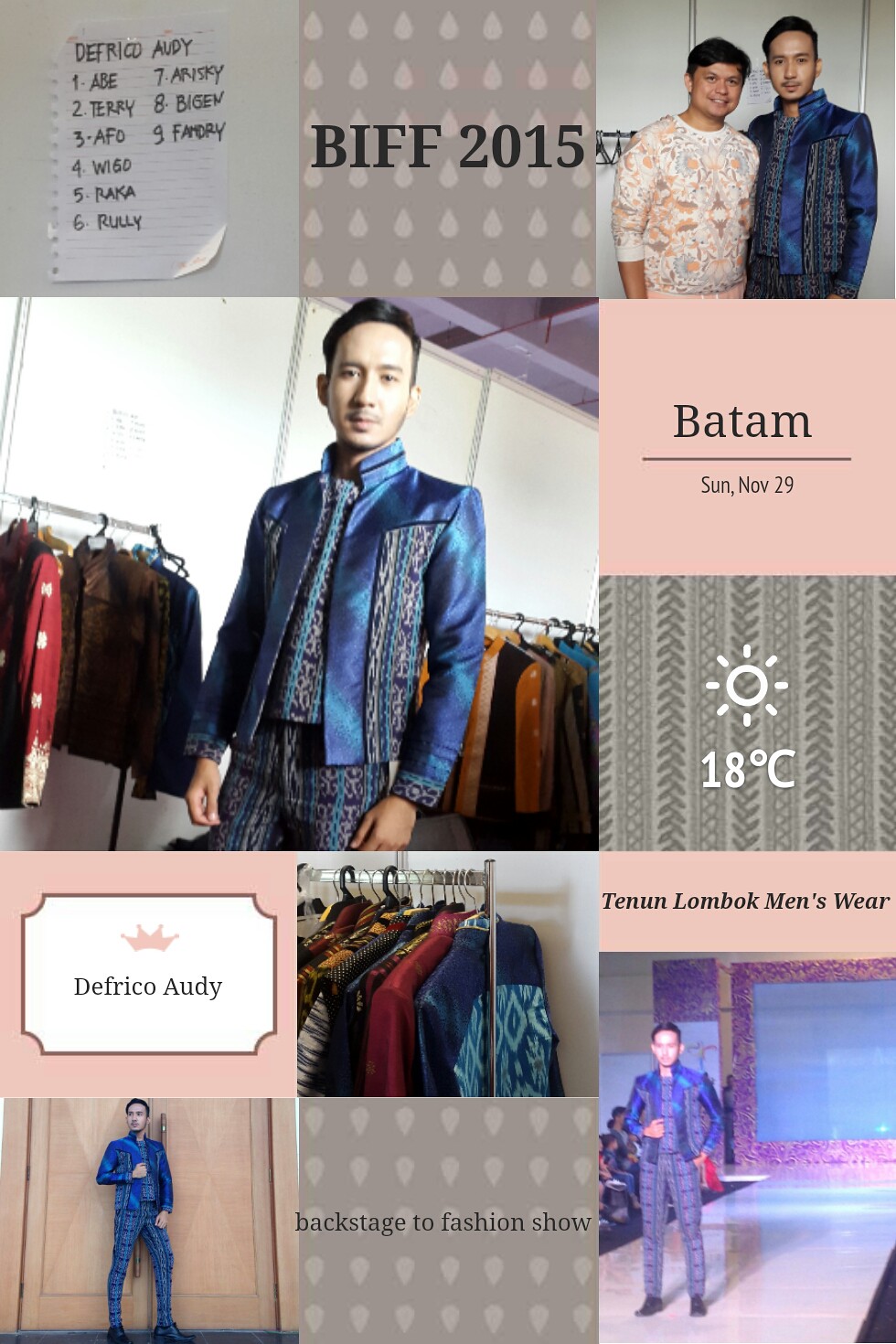This is a full-color advertisement for men's clothing, featuring a collage of various photographs. In the upper middle panel, "B.I.F.F. 2015" is prominently displayed. To the right, two young men are dressed fashionably, one in a white and orange shirt and the other in a bluish shirt. The upper left panel contains text in another language. The center of the advertisement showcases a singular young man, who seems to be a fashion model named Andy DeFrico, wearing a distinctive blue matador-style jacket with some white and purple trim, shown against a backdrop of stock jackets on racks. To the right of this image, it says "Batum, Sunday, November 29th" along with a temperature of 18 degrees centigrade, accompanied by a sun icon. Further down, the lower left panel features another image of Andy DeFrico, under the name "DeFrico Andy." The central bottom panel includes the phrase "Backstage to Fashion Show."